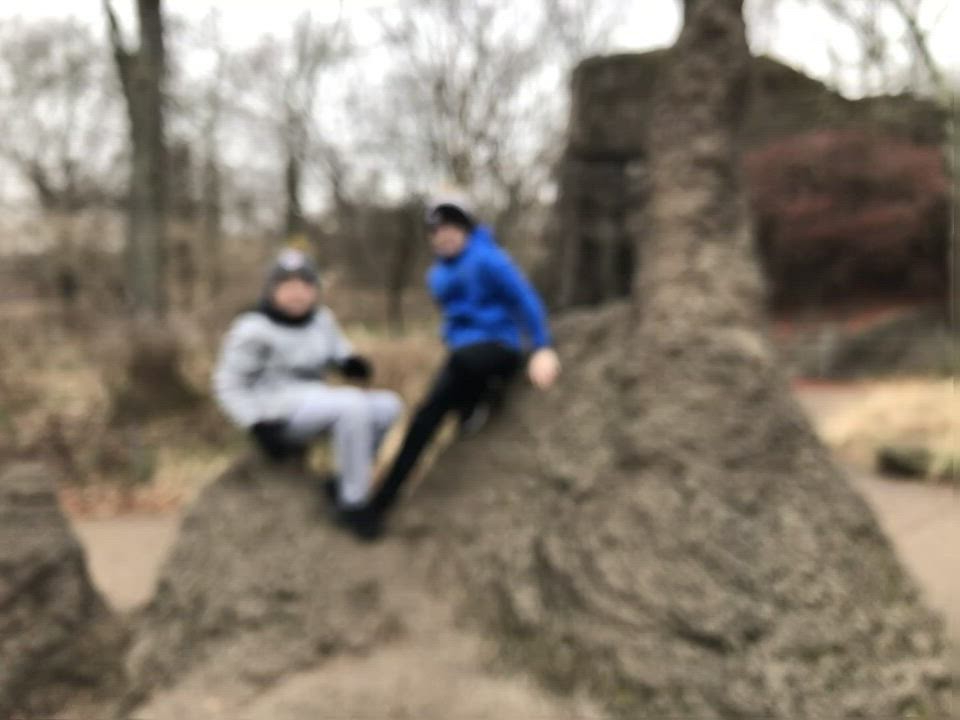In this blurred photograph, two individuals, either hikers or joggers, are seated in a serene forest setting, surrounded by nature's rugged beauty. They are perched atop a sizable rock outcropping, which dominates the foreground. The rock is a dark gray hue with lighter tan highlights, adding texture to the scene. A tall, ambiguous object—possibly another rock pillar or a tree—adds to the mystique, as the entire image is slightly out of focus.

The two figures sit in a V formation. On the left, a man sports a black beanie with a white top, a gray sweatshirt, and matching gray sweatpants adorned with writing. He completes his outfit with a scarf or neck piece, black gloves, and black shoes. On the right, the second man wears a blue sweatshirt, black pants, and black shoes. His black beanie is marked with a white symbol on the front.

Behind them, a trail weaves through the forest, flanked by trees and a prominent dark red-brown rock outcropping, adding depth to the backdrop. The photo captures a moment of rest and companionship amidst the natural ruggedness and tranquility of the forest.